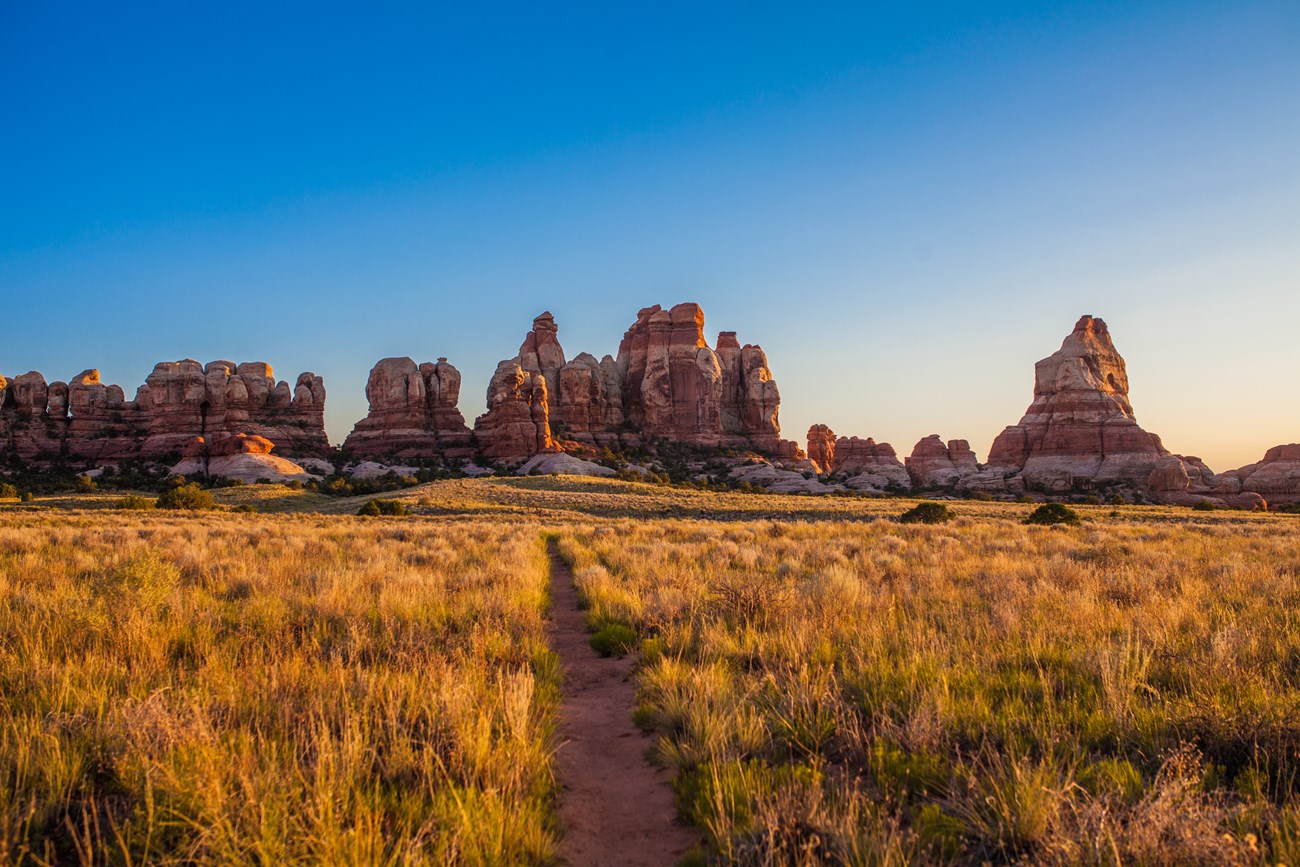This photograph captures an expansive outdoor scene dominated by a striking contrast between a vivid blue sky and an open field. The sky starts off as a clear, crisp blue at the top and softly transitions into a light peachy-orange hue near the horizon. The horizon is punctuated by a range of rugged, jagged standing stones or canyon-type rock formations featuring distinct stripes of brownish-red and white that run vertically through them. These formations are irregularly shaped, with some taking on bell-like profiles and clustered together in the middle, resembling large statues.

Beneath these towering rocks is a gradient of hills that appear white or grayish at their bases, gradually giving way to a flatter landscape of tall, green, and yellowish-brown grass. Cutting through this grassy expanse is a narrow, straight dirt pathway that extends from the foreground deep into the background, ultimately disappearing into the vanishing point. Flanking the path are a few small, brown dirt hills, which add texture to the otherwise flat terrain. The scene is serene and wonderfully captures the raw beauty of a desert or canyon-type landscape.